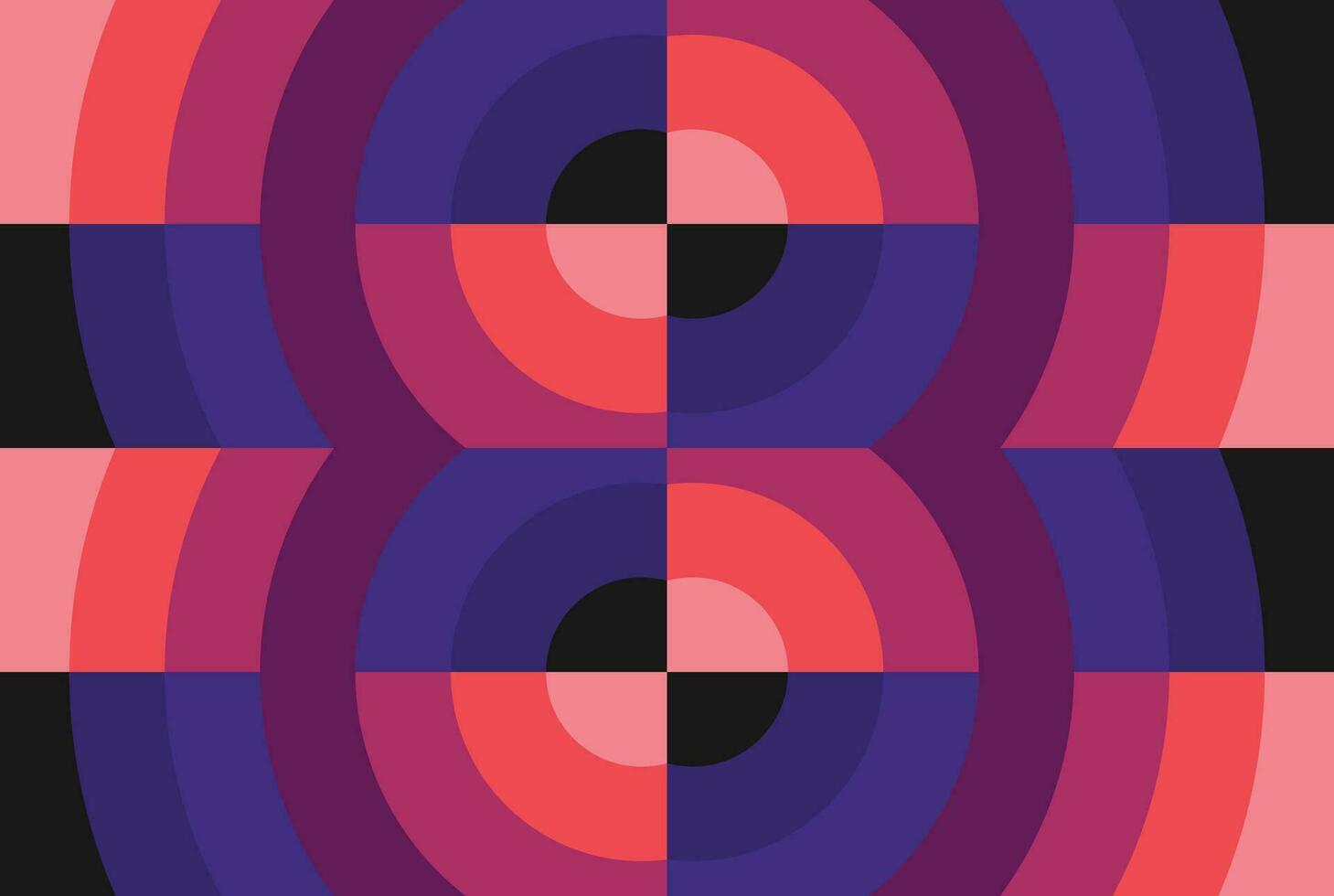The image is a highly abstract and geometrical design, evocative of art from the 60s or 70s. It's composed of two vertically stacked circles, each intricately subdivided into rectangular segments. Specifically, each circle features long, narrow rectangles set in a two-across and four-up-and-down arrangement. The circular patterns are divided radially and exhibit a vibrant array of colors including shades of pink, red, magenta, purple, blue, and black.

The design creates an intricate play with color, with each segment mixing different hues. For instance, one segment might display a pink center surrounded by neon orange, fading into darker pinks, purples, and blues, whereas another segment may feature a black center with similar color gradations. The upper circle mirrors the lower one, creating a dynamic effect of conjoined yet broken-up circles that seem to be a negative reflection of each other. Overall, this complex, multi-colored, and balanced composition blends the elements seamlessly, forming a visually captivating abstract artwork.